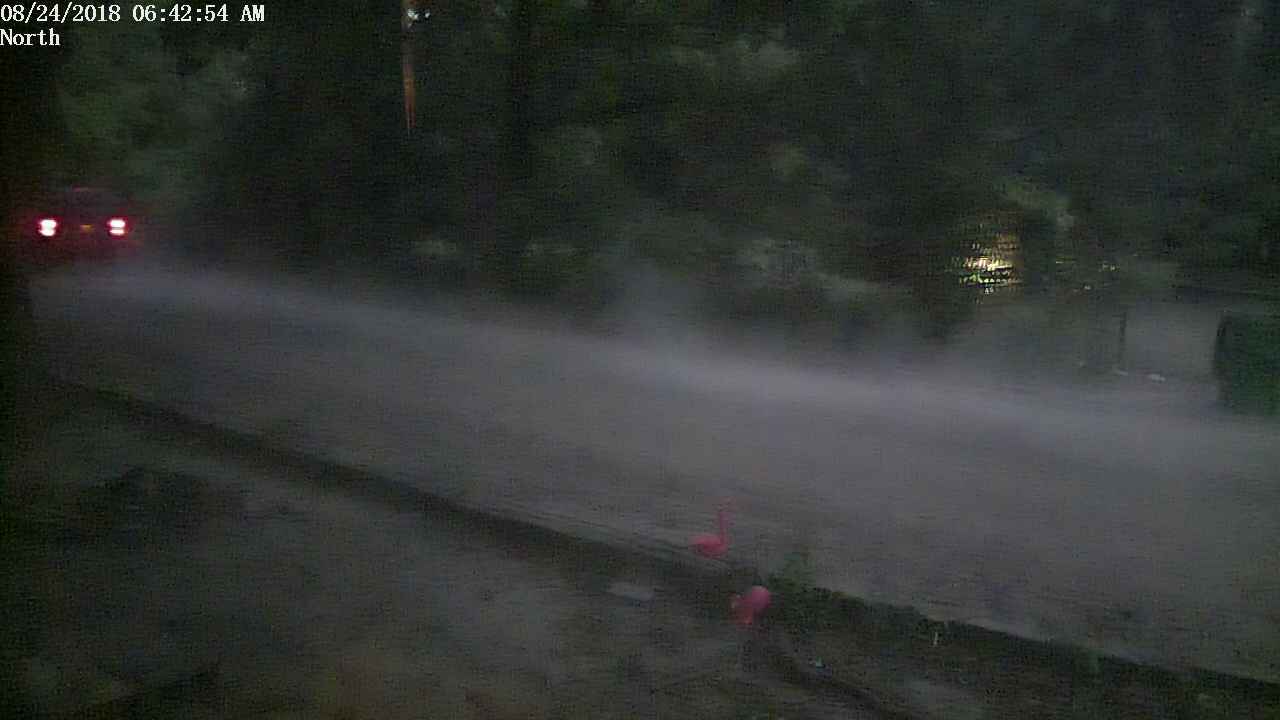Captured on August 24th, 2018, at 6:42:54 AM, this image depicts a rural dirt road with a car driving away, its taillights glowing faintly. The road, surrounded by a lush, green countryside, leads into the hazy distance where a house can be seen. The foreground is adorned with flowers resembling roses, adding a splash of color to the predominantly gray and green scene. Despite the image being somewhat blurry, the time stamp and the directional note 'north' provide a precise context.